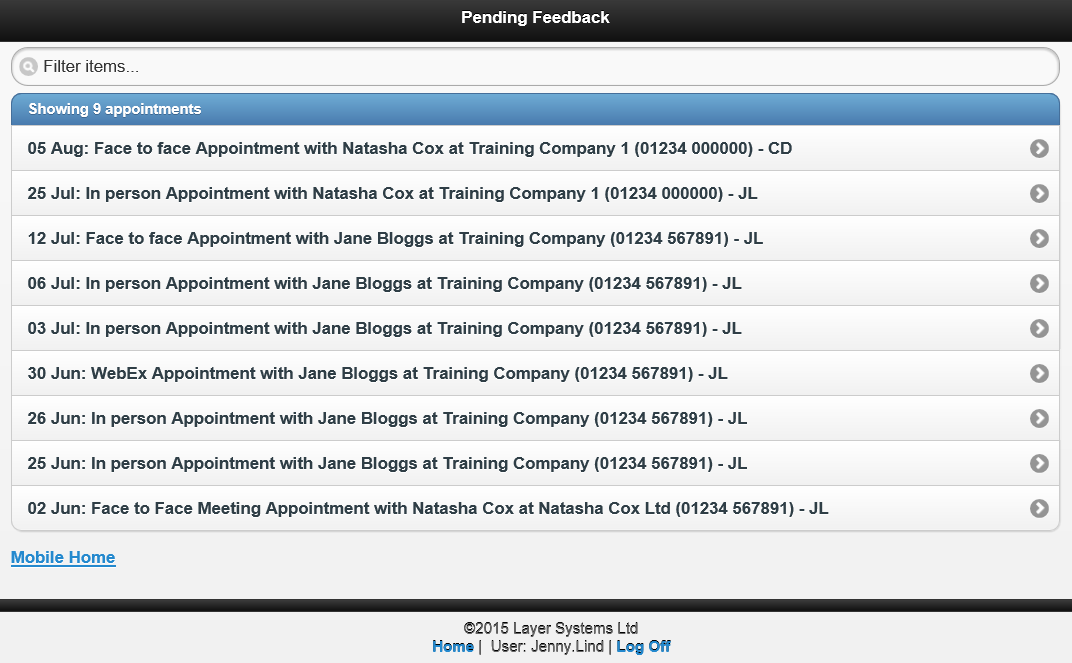This screenshot captures a section of a working system interface, highlighted by a "Pending Feedback" banner at the top against a black background with white text. Below this is a white search bar designed for filtering items. The section beneath features a title bar with a blue background that states "Showing 9 appointments," indicating the total number of entries listed.

The appointments are displayed in an expandable format, detailing various meetings: 
- A face-to-face appointment on August 5th with Natasha Cox at Training Company One.
- An in-person appointment on July 25th with Natasha Cox at Training Company One.
- A face-to-face meeting on June 2nd with Natasha Cox at Natasha Cox Unlimited.

The remaining appointments feature engagements with another contact, Jane Bloggs, also primarily at Training Company. In total, there are indeed nine appointments listed.

At the bottom of the screenshot, navigation options "Mobile" and "Home" are visible along with the user identification label "2015, Layer Systems user Jenny Lind."